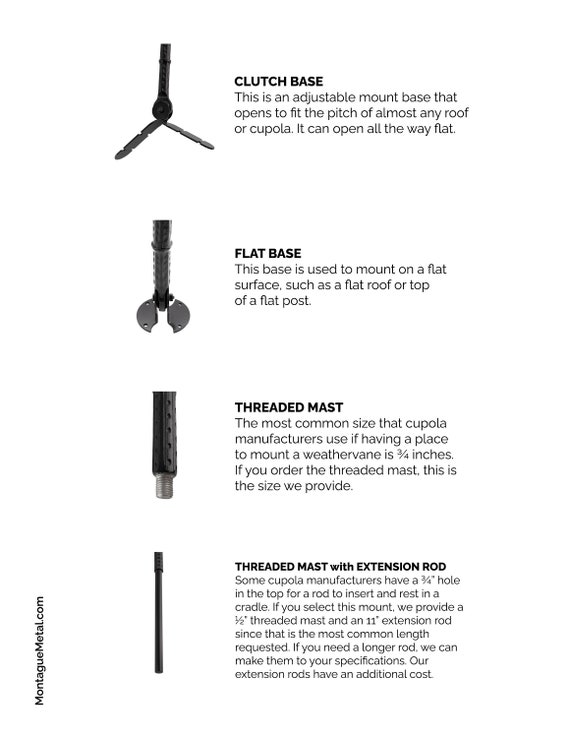This black-and-white information sheet includes four detailed images of various mounting hardware, each located on the left side, with descriptions on the right. The items, presented from top to bottom, are as follows: 

1. **Clutch Base**: An adjustable mount that opens to fit the pitch of almost any roof or cupola, capable of being fully extended to lay flat.
2. **Flat Base**: Designed for installation on flat surfaces, such as flat roofs or the tops of flat posts.
3. **Threaded Mast**: A commonly used mast in cupola manufacturing, specifically sized at 3/4 inches to accommodate the mounting of weather vanes.
4. **Threaded Mast with Extension Rod**: This mount includes a 1 1/2 inch or 1/2 inch threaded mast along with an 11-inch extension rod, offering versatility with customizable rod lengths for specific requirements, though longer rods may incur additional costs.

The descriptive text is written in a smaller, lighter font compared to the bold, all-caps titles of each item.